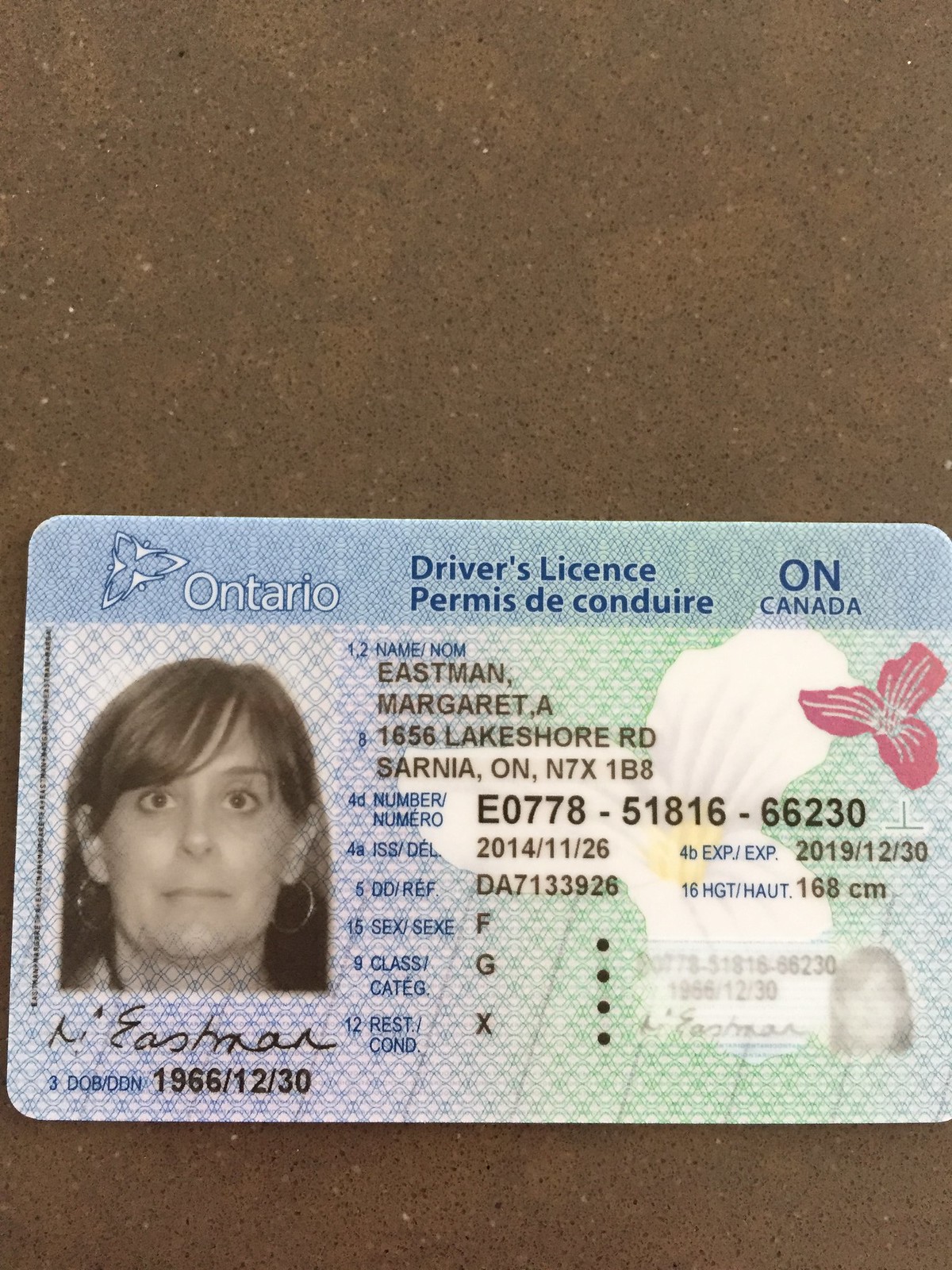This is a detailed photograph of a Canadian driver's license, specifically from Ontario, resting on a brown granite countertop. The license features a background gradient transitioning from light blue on the left to light green on the right, adorned with white and red lily patterns as part of its security design. At the top, it displays the word "Ontario" next to a triangular symbol, followed by "Driver's License" and "Permis de Conduire" in French. The far right mentions "ON" and "Canada" in blue font.

The left side showcases a black-and-white photograph of a middle-aged woman with long dark hair and gold earrings. Her details include her name, Margaret A. Eastman, her date of birth as 1966-12-30, and her address at 1656 Lakeshore Road, Serena, Ontario, N7X 1B8. The card's identification number is E0778-51816-66230, with a reference number DA7133926. It was issued on 2014-11-26 and expires on 2019-12-30. Margaret's height is recorded as 168 centimeters, and she holds a Class G license with the condition code X.